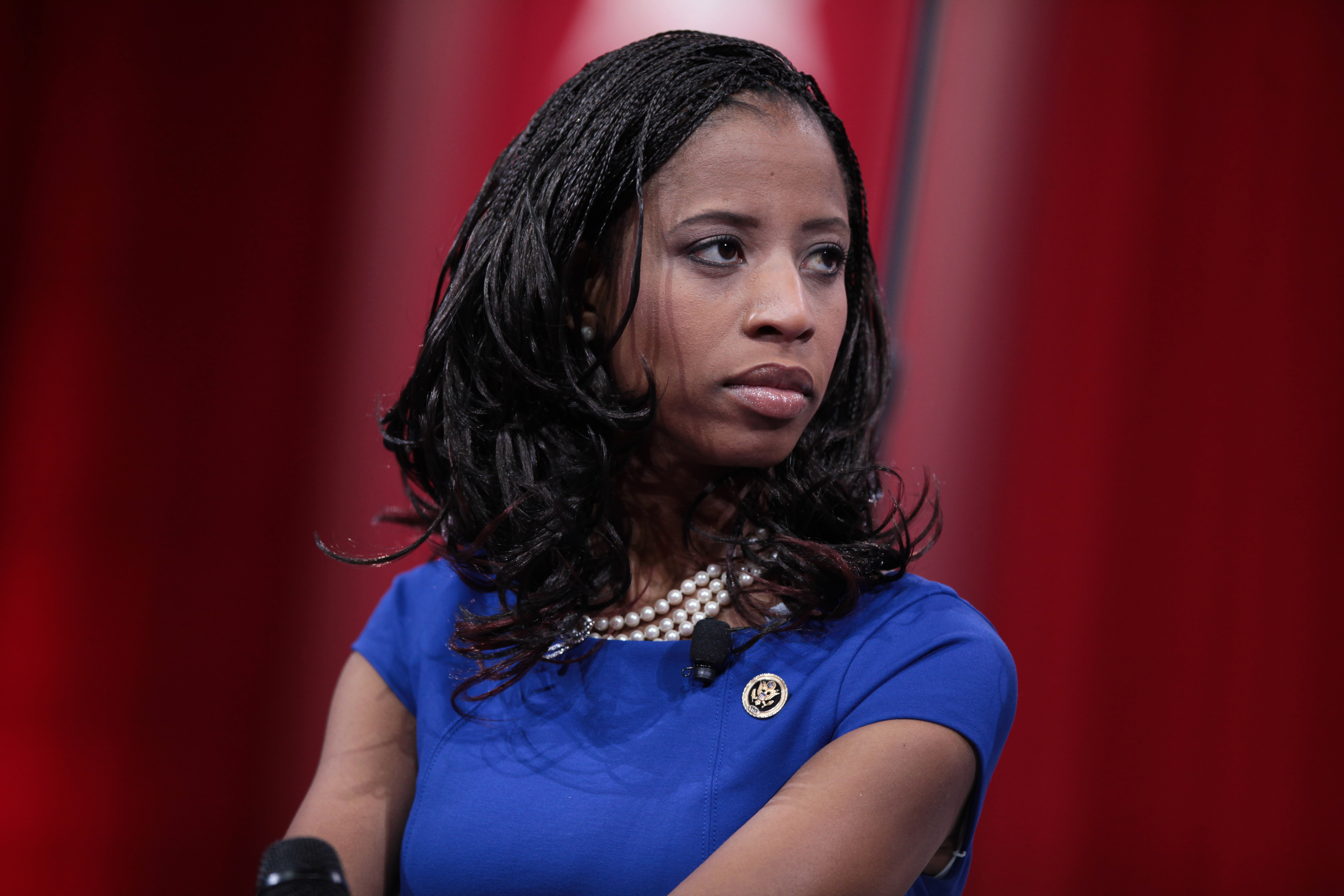The image features a detailed indoor photograph of an African-American woman who is centered and slightly turned to the right. She has shoulder-length black hair that frames her face, which is oriented slightly to the right. The woman is wearing a blue, short-sleeved top, only visible from the chest up, leaving her upper arms partly cut off at the bottom of the image. A microphone, attached to the right side of her top, points towards her face. Directly below the microphone is an emblem on her shirt. She also wears three strands of white pearls around her neck. The background is predominantly maroon, possibly a wall or curtains, but it's a bit blurry, making it hard to discern. The overall color palette includes shades of maroon, black, brown, white, pink, blue, and gold, primarily highlighted by her attire and accessories.